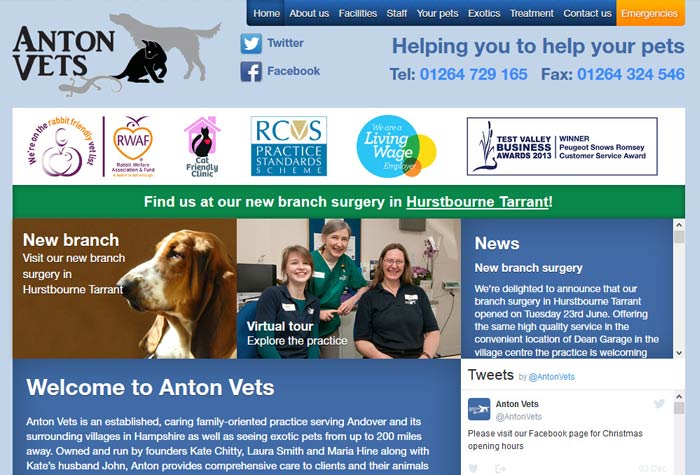This screenshot captures the homepage of Anton Vets' website, showcasing a professional and user-friendly layout dedicated to providing veterinary services.

At the top left corner, the logo prominently displays 'Anton Vets' in black letters. The logo features a black silhouette of a dog facing right, a cat positioned in front of the dog, and a gray silhouette of a lizard at the end of the cat's tail, symbolizing the range of animals they care for.

Centralized towards the top, social media icons and corresponding text for 'Twitter' and 'Facebook' provide easy access to their social channels. On the far right, the slogan 'Helping you to help your pets' is displayed in blue letters, with the clinic's telephone and fax numbers listed below for quick contact.

The top navigation bar spans from the center to the right, featuring blue buttons labeled Home, About Us, Facilities, Staff, Your Pets, Exotics, Treatment, Contact Us, and an orange-highlighted Emergencies tab, ensuring clear and easy navigation for users.

A large banner dominates the center, highlighting their achievement as the 2013 winner of the Test Valley Business Awards. Below this banner, a green strip announces their new branch surgery in Hurstbourne Tarrant.

The middle section of the page is divided into distinct content areas. On the left, a news box with a scroll bar enables visitors to browse through updates easily. On the bottom right, a tweet box allows scrolling through recent Twitter posts from Anton Vets. The bottom left features a welcome box with a blue background, introducing visitors to Anton Vets and providing an overview of their veterinary services.

Overall, the webpage is methodically structured, offering a welcoming and comprehensive overview of Anton Vets’ services and achievements to new and returning visitors alike.